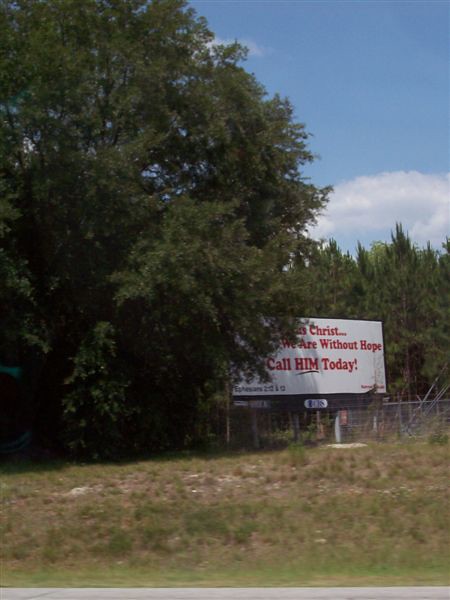This photograph captures a fleeting moment taken from the inside of a moving vehicle, evident from the slight blur in the foreground. The scene primarily consists of a grassy area featuring patches of dried grass and dirt. A metal fence runs across the image, acting as a divider between the foreground and midground. Dominating the midground is a large, white billboard adorned with red text, partially obscured by tall trees that extend upwards into the top left portion of the frame. The billboard bears a message, "Christ, we are without hope, call him today," and has a black section in the lower left corner referencing a Bible chapter. Behind the billboard, a line of tall trees stretches out, blending into a serene, flat blue sky with sparse, fluffy clouds. The billboard itself rests on the ground, not elevated.